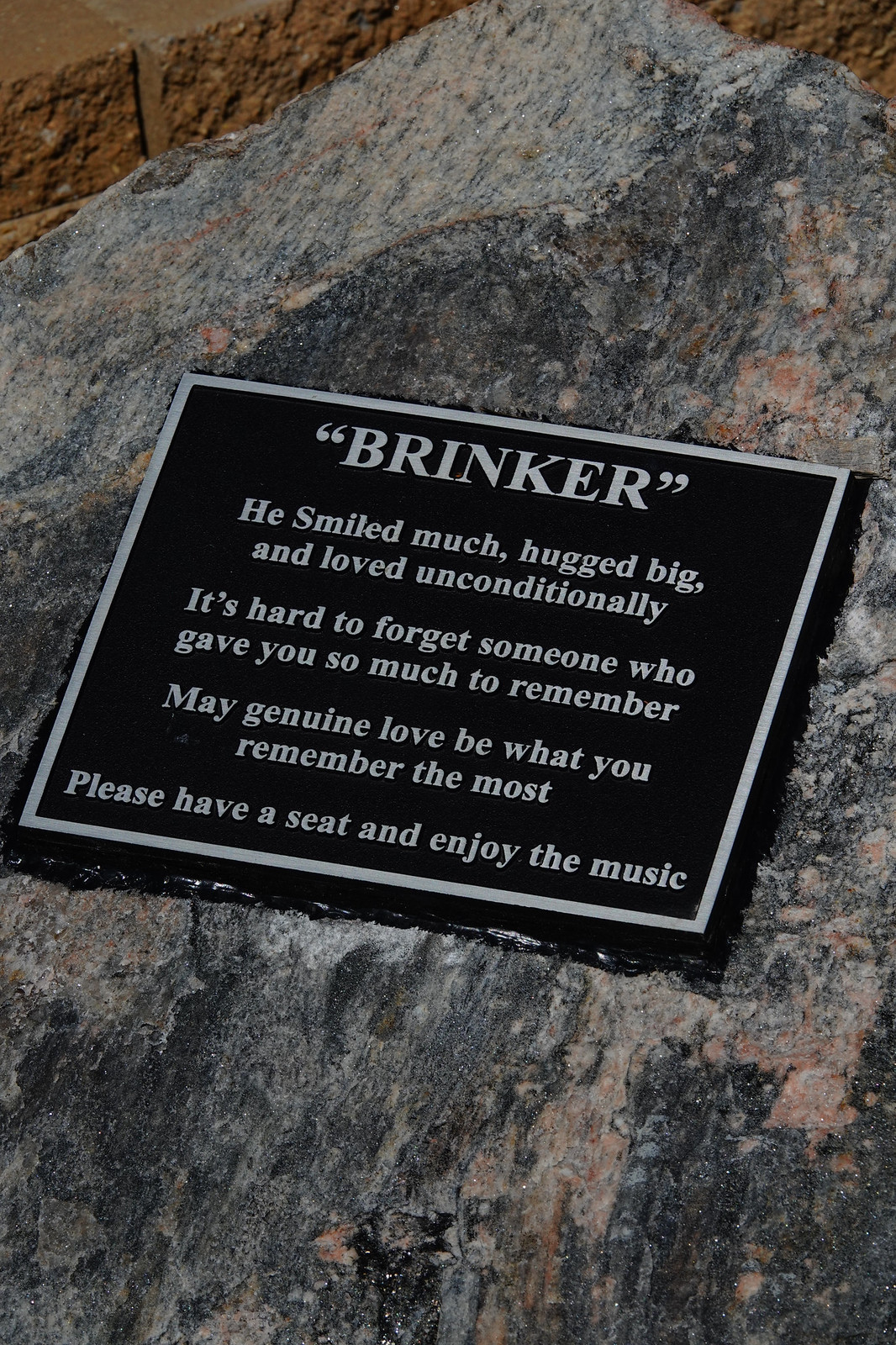The image depicts a detailed view of a black metal plaque fastened to a large rock, with a distinctive composition of black, white, and brown hues. The plaque is outlined in silver and is slightly tilted to the right. At the top, in silver quotation marks, the name "Brinker" is prominently featured. The plaque bears a heartfelt inscription: "He smiled much, hugged big, and loved unconditionally. It's hard to forget someone who gave you so much to remember. May genuine love be what you remember the most. Please have a seat and enjoy the music." Surrounding the rock, particularly in the upper left and right corners of the image, there are hints of a brown brick wall, suggesting a serene and possibly public location, such as a park or a concert hall, where visitors can sit and appreciate the music, honoring the memory of the individual commemorated by the plaque. The image is zoomed in, focusing primarily on the plaque and part of the rock, making it difficult to gauge the overall size of the rock or its surroundings.